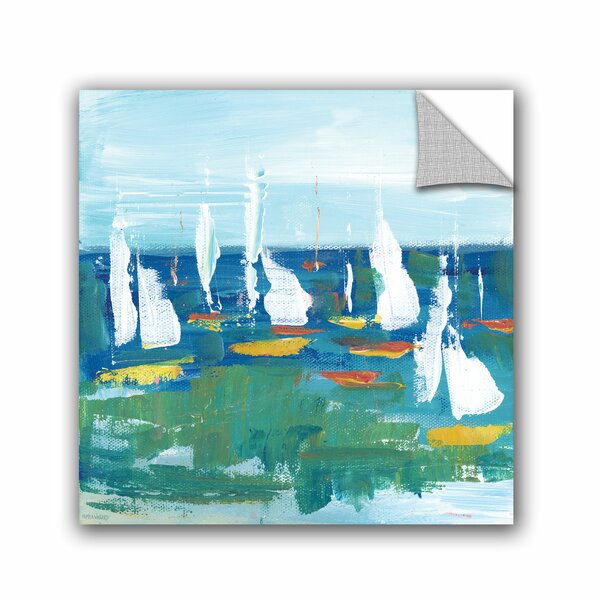The image depicts an abstract oil painting of a bustling boat harbor filled with sailboats. The water in the foreground has a greenish-blue hue, giving way to a deeper blue as it stretches toward the horizon. Various sailboats, identifiable by their white sails, float on the water with hulls painted in vivid shades of yellow, red, and orange. The painting style is characterized by thick, splotchy brushstrokes that emphasize artistic interpretation over precise detail. The sky above is a clear blue adorned with streaky cirrus clouds. Noteworthy is a unique feature in the top right corner of the image, where it appears to peel back like a sticker or a folded page in a book, adding an intriguing dimension to the artwork.